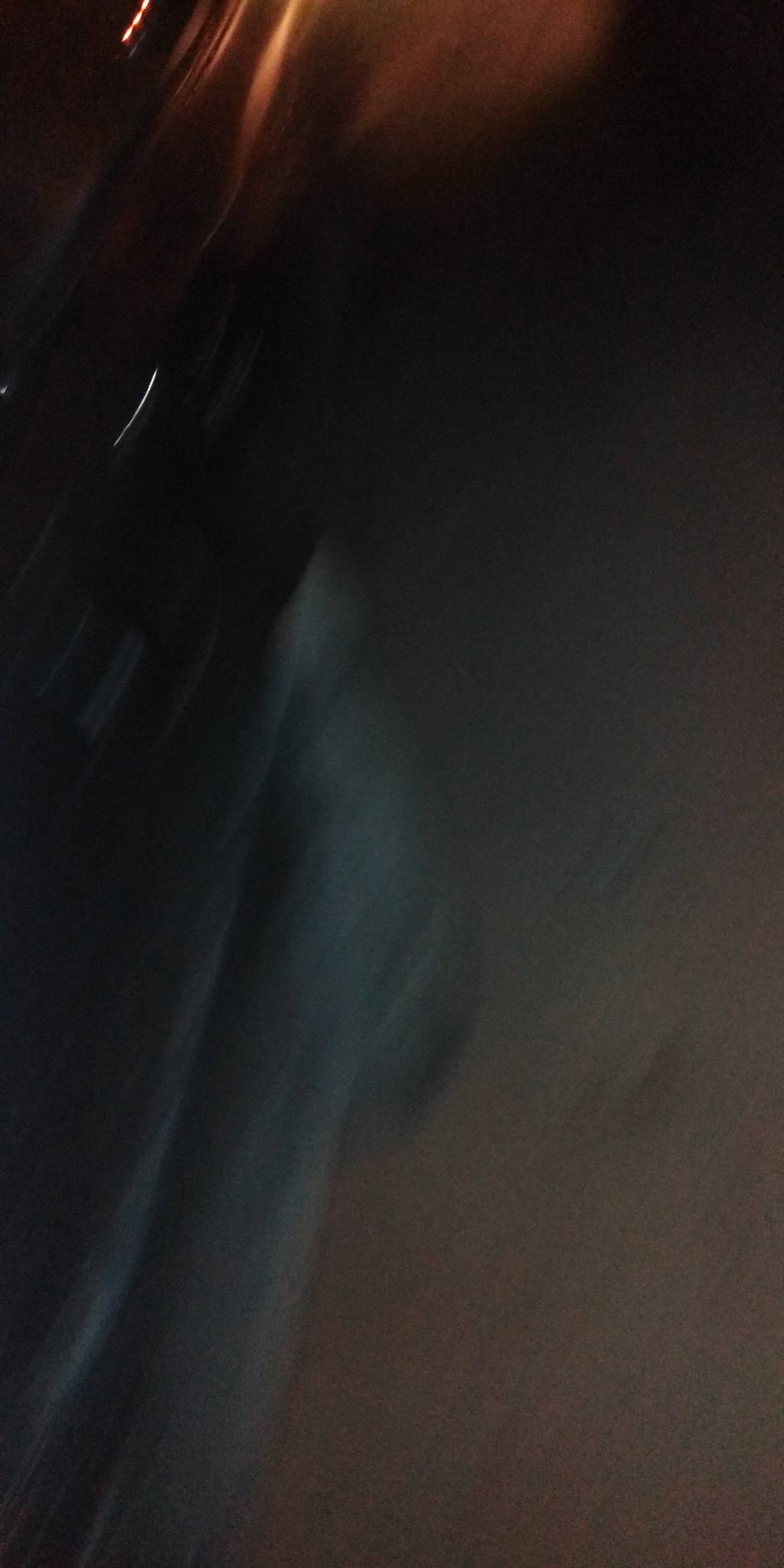This photograph appears to have been taken at night and is both very dark and blurry. At the top of the image, there are streaks of light, likely from streetlights or headlights, that have turned into elongated lines due to the motion blur. In the bottom left corner, an indistinct black shape, potentially a car, extends from the lower left towards the center of the frame. The entire right side of the image is a grayish tone, which might represent a road surface. The image orientation seems to be rotated, suggesting that the right side should be the bottom and the left side should be the top. Additionally, there is a shaded area on the black object resembling a car tire, hinting at the presence of a vehicle.